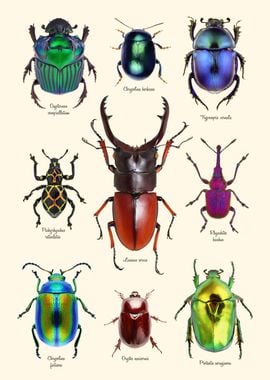This image appears to be a detailed diagram from a book, showcasing nine labeled scarab beetles arranged on a cream-colored stock page. The beetles, organized in three rows and three columns, exhibit a broad spectrum of vibrant colors and intricate patterns, though the small black font labels beneath each beetle are difficult to read.

Starting from the top row, the first beetle on the left is a wide, short metallic green with black abdominal marks, a black head, and six black legs. The middle beetle in this row is smaller, rounded, black with bluish-green markings. The third beetle on the right is primarily blue with a divided back and some black accents.

In the second row, the left beetle is dark brown, sporting yellow-outlined diamonds on its back. The central beetle, possibly a Goliath beetle, is notable for its large red lower half, black upper body, and red-tinged legs. The right beetle in this row is a purplish-red with blue markings.

The bottom row begins on the left with a beetle resembling a metallic June bug, displaying a blue-green-gold sheen. The middle beetle here is medium brown and slightly smaller than its neighbors. The rightmost beetle transitions from green to yellow, featuring a brown center.

Despite the inability to clearly read the labels, the diverse array of shapes, sizes, and metallic shades emphasizes the rich variety within this collection of beetles.